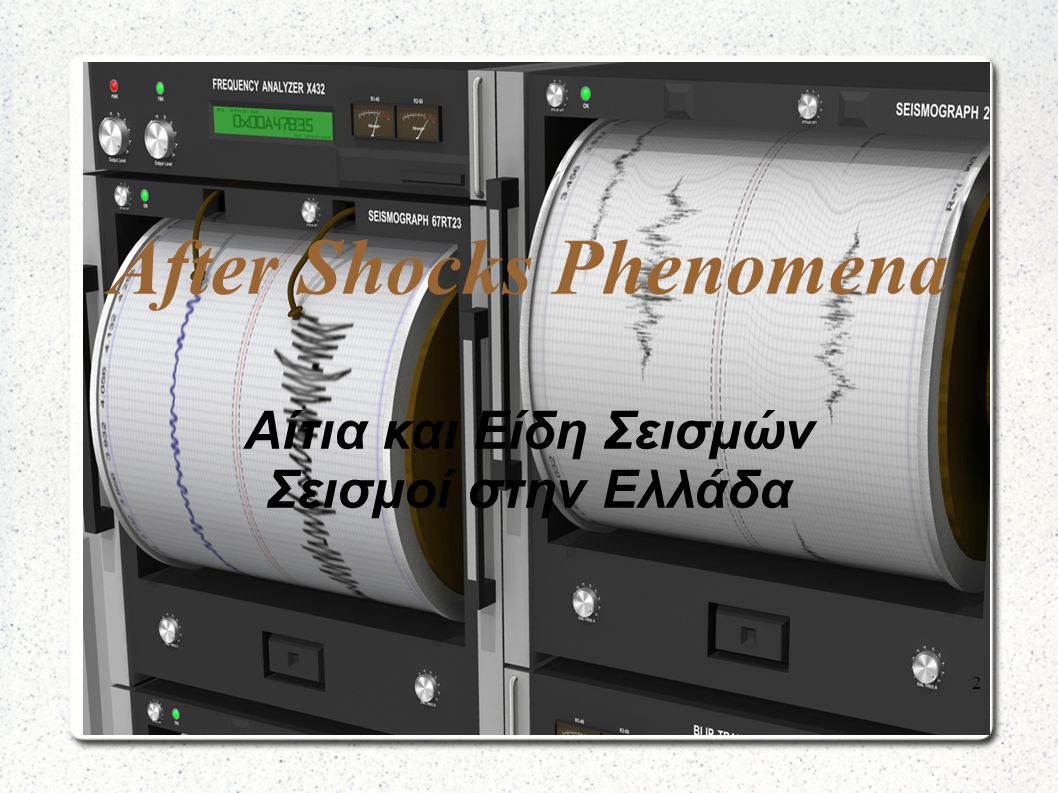This image showcases two adjacent seismograph machines with numerous intricate details. Both machines are primarily black with some white print and feature various texts and buttons. The left machine has a label at the top that reads "Frequency Analyzer X432" beneath which lies a rectangular green digital screen. The right machine, similarly structured, has the text "Seismograph 67RT23" on the upper right corner above the paper output.

Both devices are equipped with green buttons next to silver ones, likely power buttons. At the upper right corner of each, just above the paper rolls, we see squiggly seismographic lines in different colors—blue on the left and black on the right, with the right one exhibiting larger lines.

Prominent black bold print spans the center of both machines, comprising foreign text that readers cannot decipher. Above this foreign text, a title in light brown font reads "Aftershock Phenomena." Surrounding these machines is a white border with a speckled gray or white square background.

The seismographic chart recorders not only depict post-seismic activity through their detailed recordings but present a confluence of varied linguistic details, enhancing the complexity and scientific context of the image.